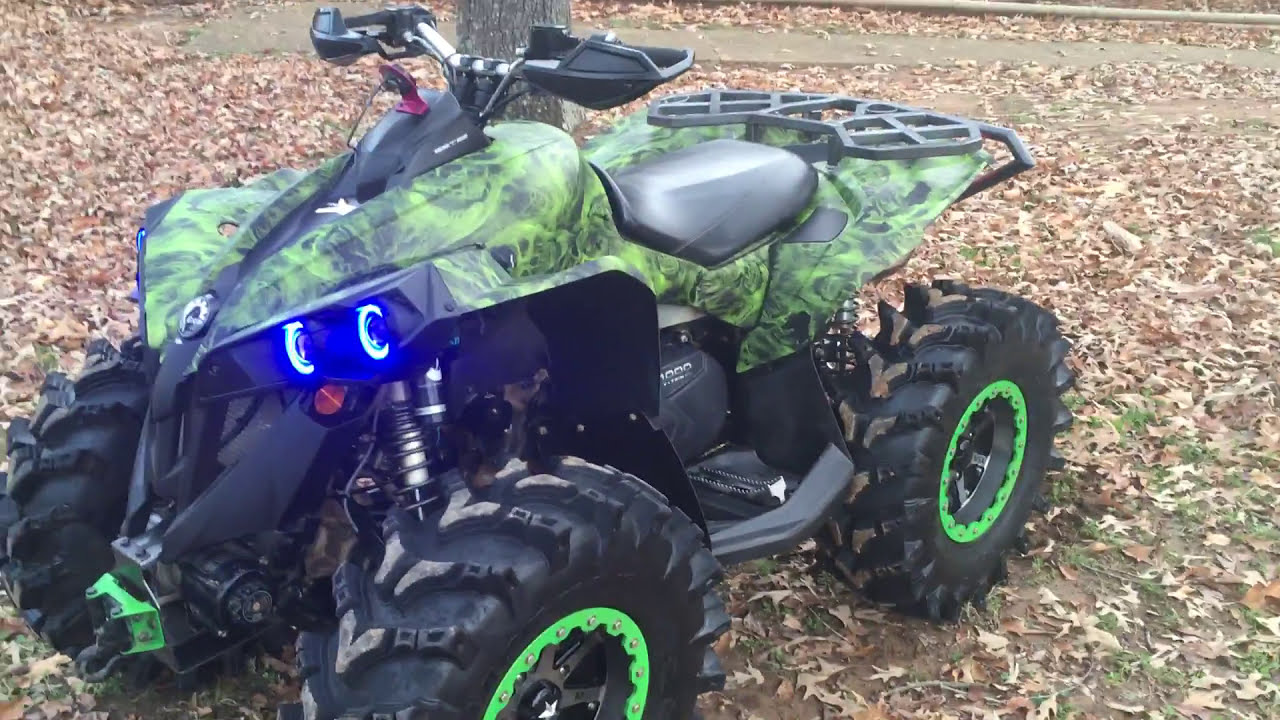The image showcases a green camouflage all-terrain vehicle (ATV) parked in an outdoor fall setting. The vehicle, which currently has no rider, features prominent green rims on its black tires, a black seat, and striking blue LED headlights. It has silver and black handles and a green mount with a black towing hook on the front. On top of the ATV, a red key is visible. The ATV is positioned on a ground covered with dead brown leaves, suggesting it is autumn. The setting also includes a flat area with a brown tree behind the ATV and a cement sidewalk further back. The overall scene captures the essence of an ATV ready for exciting rides in a picturesque fall landscape.